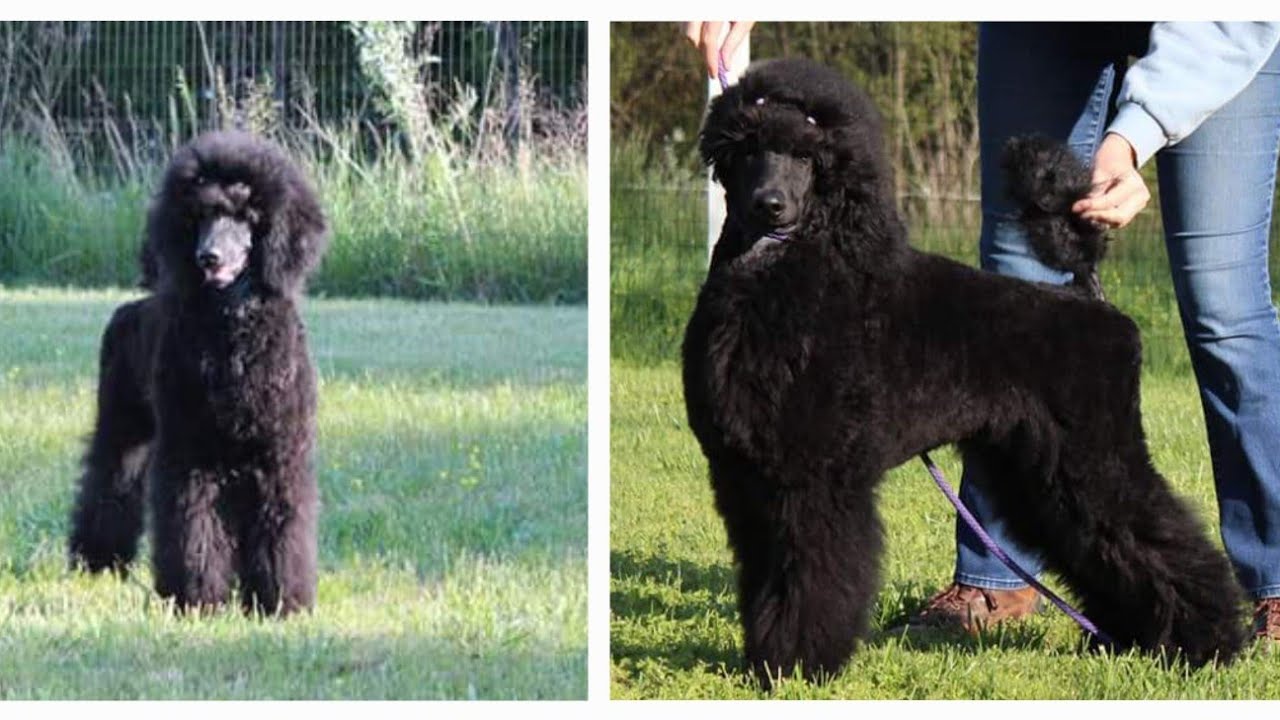This is a color landscape photo split into two distinct images by a white dividing bar. Both images feature a black poodle, likely the same dog. On the left, the poodle stands alone in a grassy area with taller grass and a wire fence in the background. The image is slightly blurred and has a vintage feel, showing the dog facing forward with its mouth slightly open. On the right, the poodle stands in a clearer, more modern photo facing left but with its face directed towards the camera. A person, visible only from the waist down and dressed in blue jeans, brown shoes, and a long-sleeved sweater, is behind the dog. The person's left hand is holding the dog's tail up, while the right hand, possibly holding a brush, is grooming the dog's head. The dog also has a purple leash on, and similar grassy terrain and fencing can be seen as in the left image.